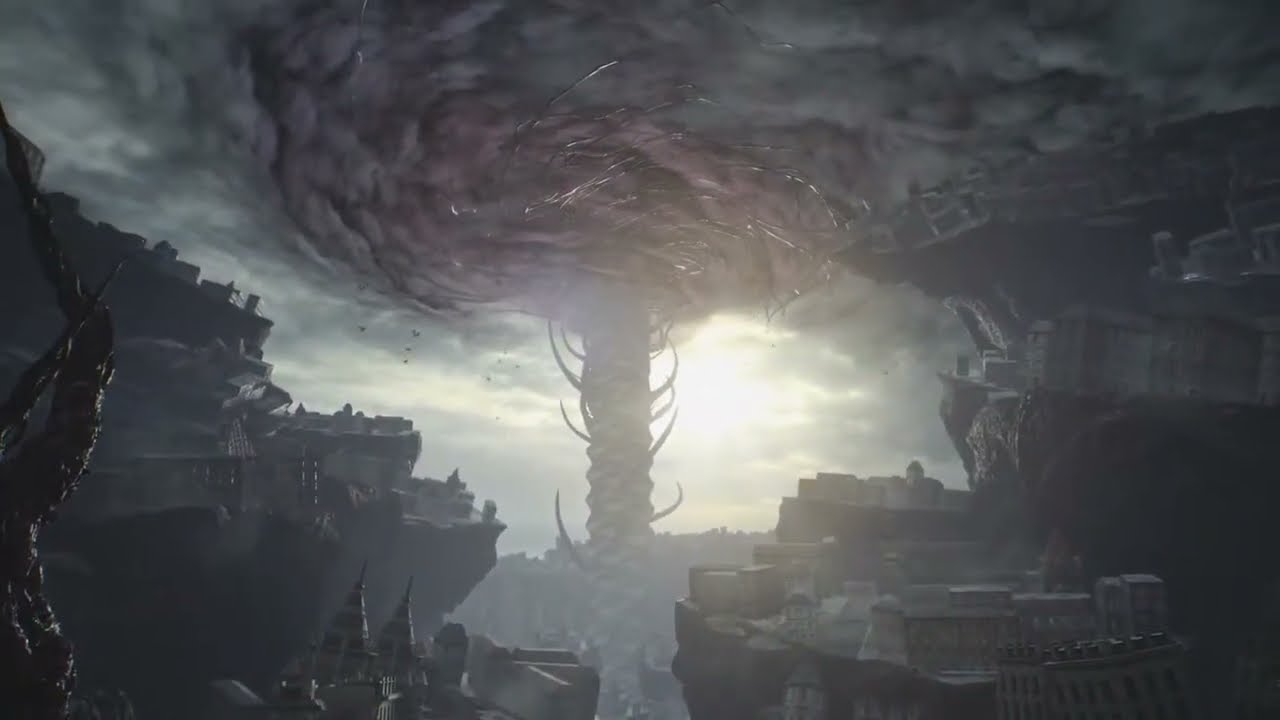This rectangular, horizontal image, possibly a screenshot from a video game, depicts a dystopian scene characterized by ominous, swirling clouds at the top that resemble a tornado or twister. The sky exhibits a range of colors from gray and black to some purples and hints of bright, white sunlight breaking through in the background. 

Centered within the image, descending from the swirling clouds, is a bizarre cylindrical stalk adorned with sharp, claw-like tendrils, suggesting a creature or an unnatural formation. The stalk appears to root itself in the ground below, adding to the unsettling atmosphere. Flanking this central stalk are two rocky cliff ledges that extend from the top towards the middle of the image. These ledges, layered and rugged, support an assortment of buildings, which exhibit a mix of architectural styles reminiscent of ancient Greek and Roman times. Some of the structures appear almost haphazardly perched on the cliffs.

In the lower left corner, an old, gnarled vine without leaves adds to the scene’s eerie nature. The overall color scheme of the image is dominated by shades of gray, white, and black, contributing to its stark, dystopian feel. The absence of characters and the dramatic, swirling sky enhance the sense of desolation and tension in this mysterious world.